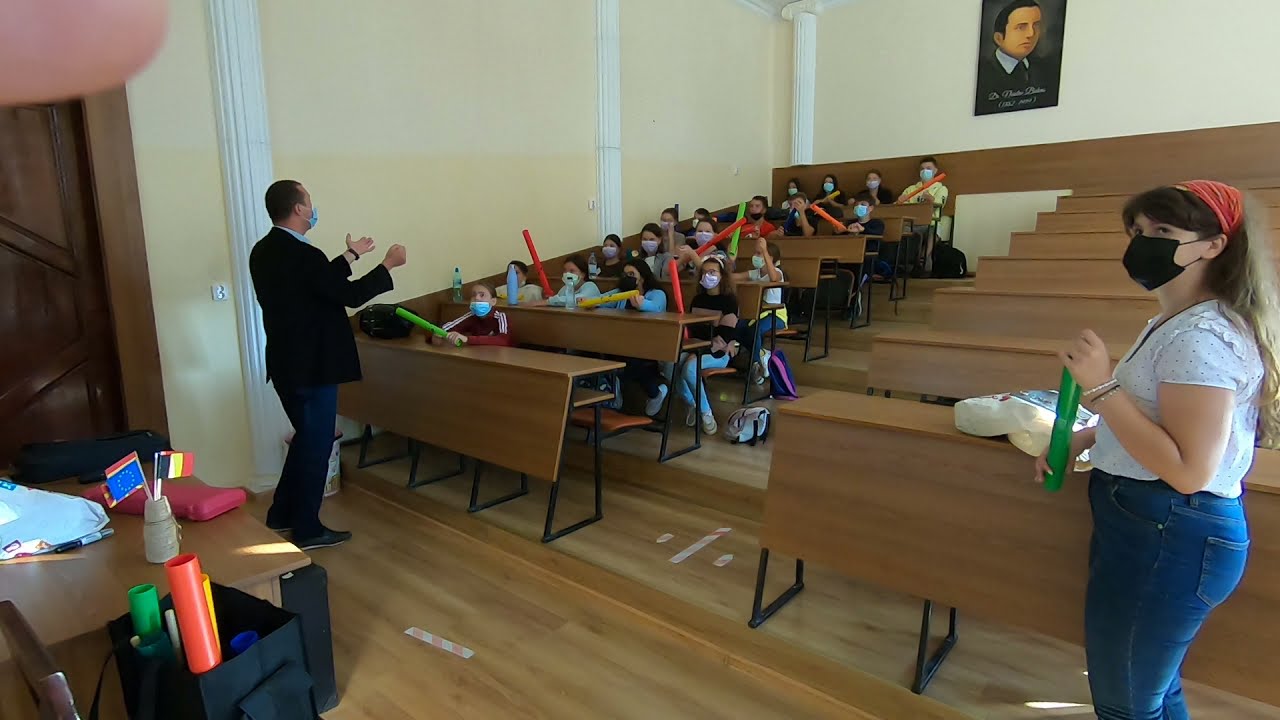The image depicts an indoor classroom setting during the daytime. The room features light beige walls and wooden floors, and it is arranged with raised levels incorporating long wooden benches and chairs. On the right side of the image, there is a woman of Caucasian descent with long brown hair, pulled back with a red bandana, and some short bangs. She is wearing a black face mask, a short-sleeved light-colored polka dot shirt, and blue jeans. The woman is holding a green cylindrical object, resembling a pool noodle. To the center-left and extending to the background of the image, rows of children are seated on the benches. They also hold colorful cylindrical objects—green, red, blue, and yellow—and most of them are wearing face masks. Facing the children is a man of Caucasian descent, dressed in a black dress jacket and blue jeans, and wearing a blue face mask. Above him, on the back wall, hangs a rectangular picture of a man in a black suit. The lower left corner of the image shows a desk filled with various classroom items, while the upper left corner reveals what appears to be the back of someone's thumb, slightly out of focus.